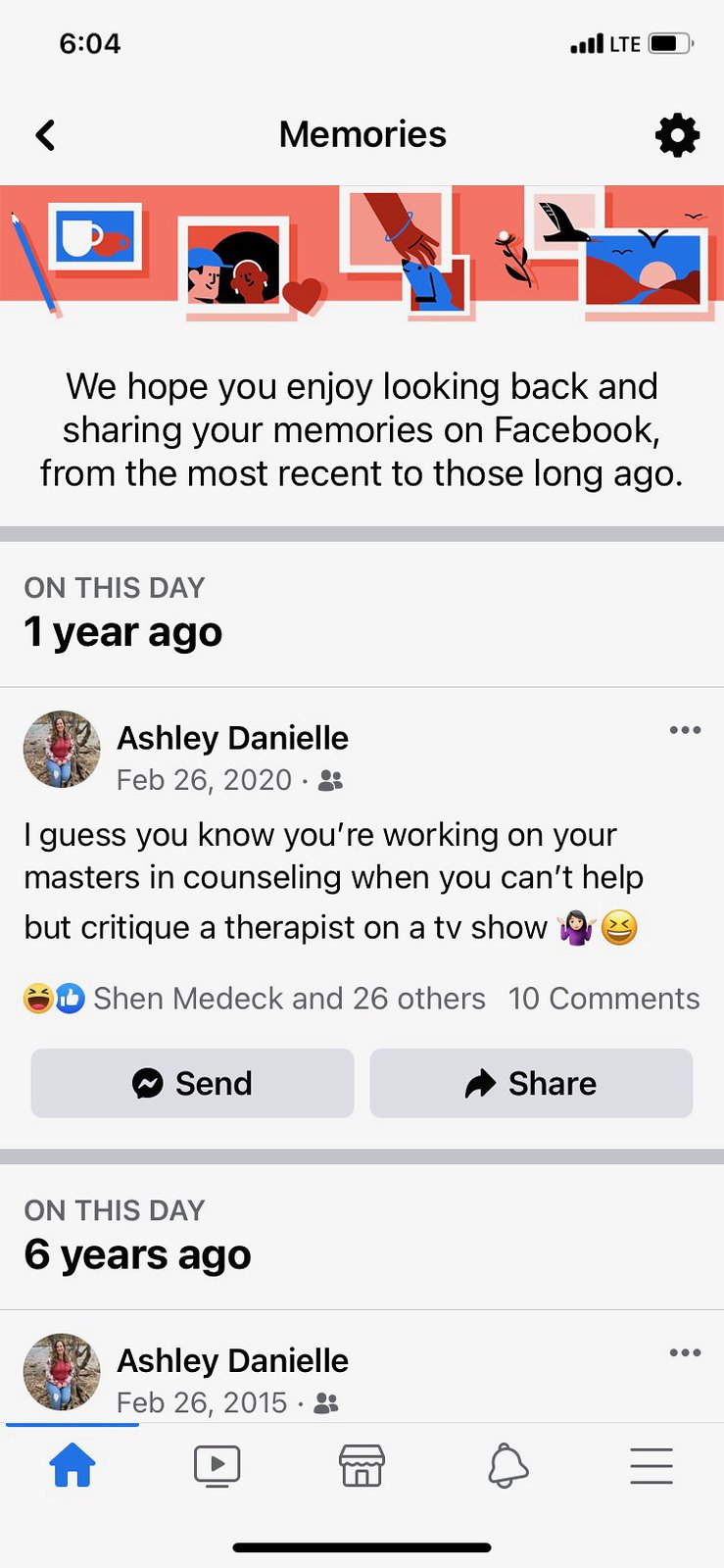The image is a grayscale screenshot of a smartphone displaying a Facebook app's "Memories" section. At the top of the screen, the time reads 6:04 with typical status icons: LTE signal strength at maximum and a battery indicator showing around 75-80% remaining. Below this, "Memories" is written in black on a gray background, accompanied by a navigation arrow. There’s a red border with six abstract images, including a couple hugging, a hand, and a seashore. 

The text below this border reads, "We hope you enjoy looking back and sharing your memories on Facebook, from the most recent to those long ago." Beneath, "On this day" in bold is followed by "one year ago," with the icon and name, Ashley Danielle, and the date, February 26, 2020. The accompanying message humorously notes, "I guess you know you're working on your master's in counseling when you can't help but critique a therapist on a TV show," adorned with a smiley face emoji. The post received thumbs-up reactions from Shen Medek and 26 others, along with 10 comments.

Further down, another note marks an event "on this day six years ago" with similar details about Ashley Danielle from February 26, 2015. The bottom of the screen features app navigation icons: a highlighted home button, a video icon, a shopping-like hut icon, a bell, and a menu represented by three horizontal lines.